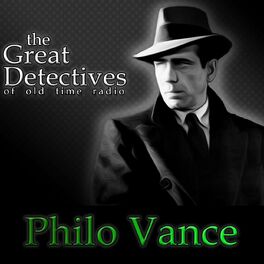The image depicts a serious-looking man, dressed as a classic detective, set against a predominantly black background. He is attired in a black trench coat, a white collared shirt with a black tie, and a wide-brimmed black hat. The man, who resembles Humphrey Bogart, is positioned with a white halo of light behind him, creating a stark contrast. The image appears illustrative rather than photographic, enhancing the vintage detective aesthetic. On the left side, white text reads "The Great Detectives of Old Time Radio," while at the bottom, in larger green font, the name "Philo Vance" is prominently displayed. The overall composition gives the impression of an old-time radio show or a retro movie cover.